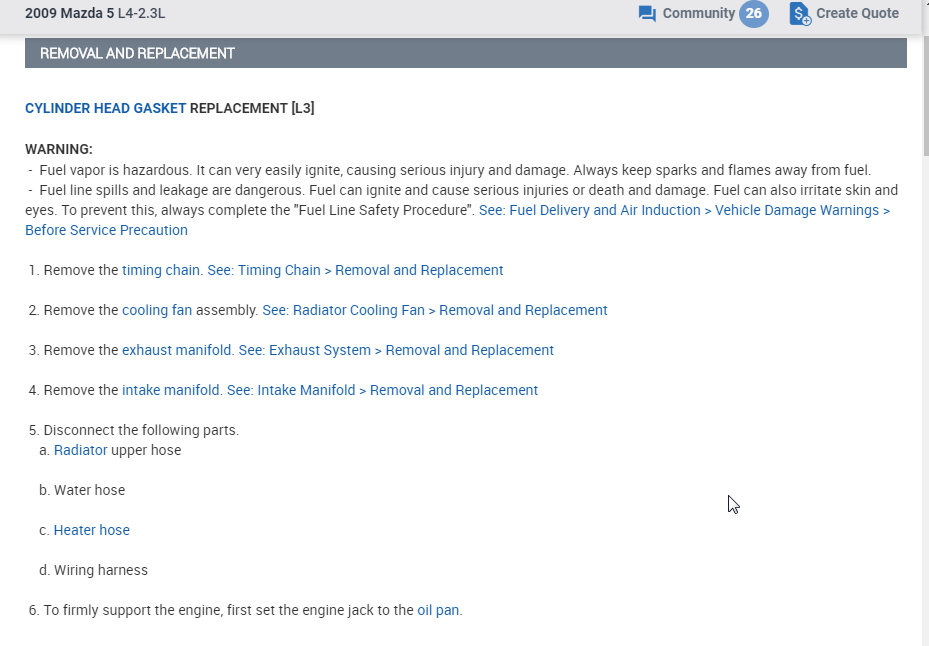This detailed instructional page outlines the process of removing and replacing the cylinder head gasket on a 2009 Mazda 5 L4-2.3L vehicle. The title of the page, set against a gray background, reads "2009 Mazda 5 L4-2.3L - Community 26: Create Quotes, Removal and Replacement, Cylinder Head Gasket Replacement." "Removal and Replacement" is highlighted with dark gray background and white text, while the rest of the page has a white background with black text. Certain parts of the text appear in blue, indicating clickable links leading to additional resources.

The page contains a critical warning highlighting the dangers of fuel vapor, which can easily ignite, causing severe injuries, death, or significant damage. It stresses the importance of keeping sparks and flames away and urges the reader to always follow the fuel line safety procedure for fuel spills and leakages, as outlined in the "Fuel Delivery and Air Induction" and "Vehicle Damage Warnings" sections.

The procedure to replace the cylinder head gasket begins as follows:

1. **Remove the Timing Chain:** Refer to the "Timing Chain Removal and Replacement" section for detailed steps.
2. **Remove the Cooling Fan Assembly:** Instructions are provided in the "Radiator Cooling Fan Removal and Replacement" section.
3. **Remove the Exhaust Manifold:** Detailed steps can be found in the "Exhaust System Removal and Replacement" section.
4. **Remove the Intake Manifold:** Consult the "Intake Manifold Removal and Replacement" section.
5. **Disconnect the Following Parts:**
   - a. Radiator upper hose
   - b. Water hose
   - c. Heater hose
   - d. Wiring harness
6. **Firmly Support the Engine:** Begin by setting an engine jack under the oil pan for support.

All these steps are meticulously designed to guide users through the process of replacing the cylinder head gasket on the specified 2009 Mazda 5 L4-2.3L model. The page serves as a comprehensive manual for what appears to be a minivan.